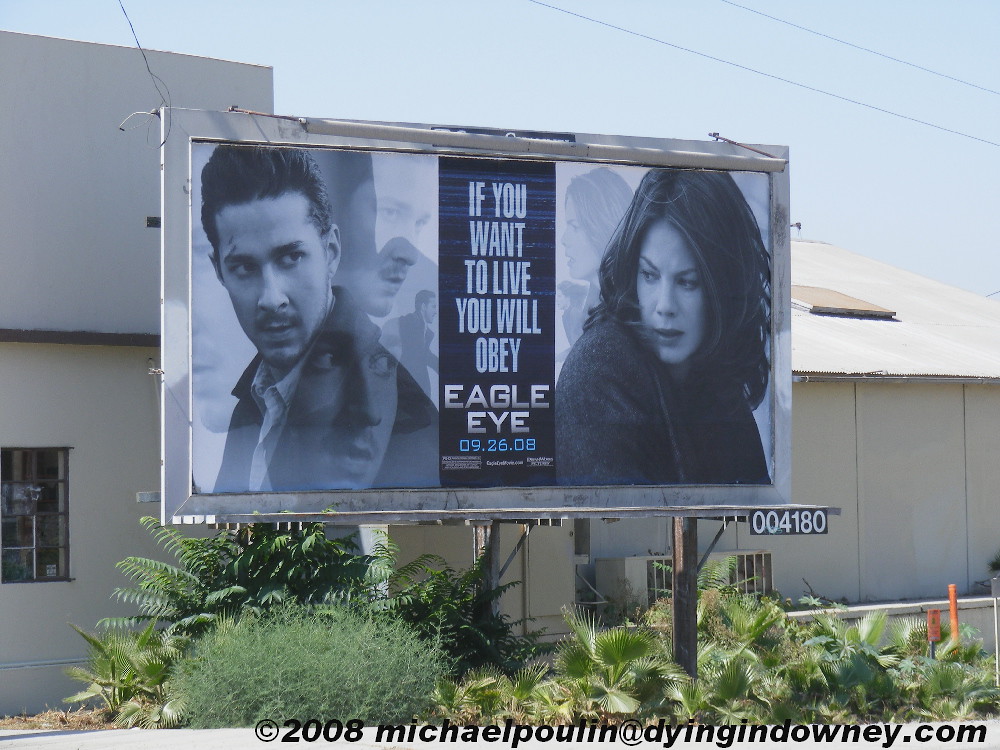In this photograph, a billboard is prominently displayed in the center, slightly angled so the right side recedes behind the left. The billboard, framed in gray, features a light gray-blue background with a central dark rectangle. The dark rectangle, adorned with faint horizontal blue lines, bears the following message in light blue all-cap letters: "IF YOU" followed by "WANT," "TO LIVE," "YOU WILL," and "OBEY" each on a new line. Below, "EAGLE" is written in white and underlined by "I" in light blue. Beneath that, in light blue, the date "09.26.08" is indicated. Additionally, the billboard subtly displays superimposed images of a woman with dark, shoulder-length hair wearing a dark sweater on the right, and a man with short dark hair dressed in a dark jacket and a light button-down shirt on the left, giving the appearance of their faces lightly blending into the background. Behind the billboard, a white and gray building stands, while green fern-like plants are seen below. The sky overhead is a light gray-blue, completing the scene.